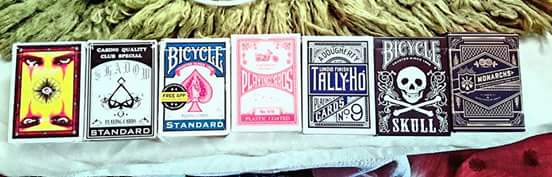Displayed on a shelf beneath a shaggy, woolen fringe are seven rectangular items, which appear to be packs of playing cards. Each pack is in pristine condition, and they showcase a variety of designs and colors. Starting from the right, the first two packs are black and white; one features a skull and crossbones motif. The third pack, in blue and white, confirms they are indeed playing cards. Positioned centrally, the fourth pack is pink and white, although its details are slightly out of focus. The fifth pack is blue with a red spade symbol and is labeled "Bicycle Standard." The sixth pack is in black and white and also bears the "Standard" label. Lastly, the seventh pack on the far left stands out with its unusual design: a yellow background with a maroon and black border, adorned with two sets of eyes—one pair looks directly at the viewer from the top, while the other, at the bottom, gazes upward towards the center, along with an enigmatic symbol.